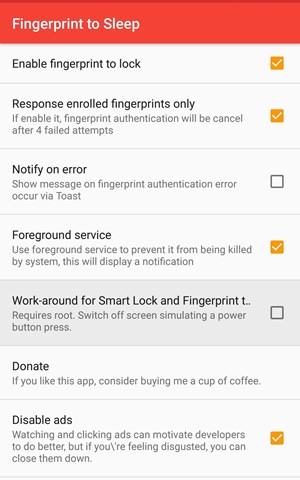This image captures a settings tab labeled "Fingerprint to Sleep," featuring various configuration options for fingerprint-enabled functionalities. On the left, a series of checkboxes indicate the status of each setting:

1. "Enable fingerprint to lock" is activated, indicated by an orange checkmark inside a white arrowed box.
2. "Response to enrolled fingerprints only" is also activated, with a description beneath it.
3. "Notify on error" remains inactive, its checkbox empty.
4. "Foreground service" is enabled, complete with a descriptive line underneath.
5. "Workaround for smart lock and fingerprint" is listed, but its checkbox is not selected. The text following it starts with a 'T' but is truncated and unreadable; a description is provided below.
6. The word "Donate" is evident, accompanied by a description, though without an associated checkbox.
7. Lastly, "Disable at" is enabled, its checkbox filled.

Each option is carefully listed with their respective activation status, providing a comprehensive view of the fingerprint lock settings on this device.